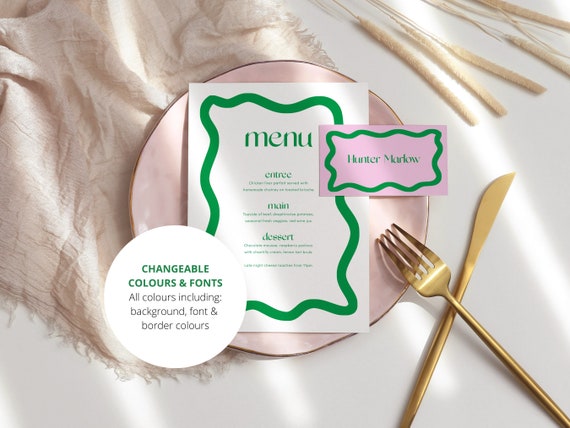The image showcases a close-up of a minimalist and neatly arranged table setting on a white tablecloth. At the center is a pink plate, which holds a small menu adorned with a green squiggly border. The menu is simple, categorized with titles such as Entree, Main, and Dessert, but the specific descriptions underneath are not legible. Adjacent to the menu, a rectangular name tag with a similar green border reads "Hunter Marlowe." Below on the menu, a circle clearly identifies the text “Changeable Colors and Fonts,” hinting at an editable or customizable menu design typically offered by a menu design site.

A golden fork and knife are artfully crossed like an X at the lower right corner of the pink plate. Behind the plate, an aesthetically placed bunch of cattail-like plant pieces adds a rustic touch. The overall view is softened further with a beige handkerchief beneath the plate. The setting is dappled with light filtering in columns, adding depth and focus to the table’s arrangement, while parts of the scene remain in shadows, creating a calm and inviting atmosphere.